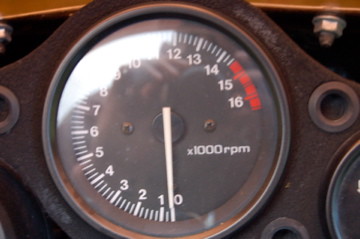This compact rectangular photograph prominently features a tachometer, its details capturing immediate attention. The tachometer forms the central element of the image, housed within a dark brown-gray, metal-like frame. Visible fastening components—specifically bolts and nuts—secure the tachometer at both the upper right and upper left corners, depicting a sturdy installation. The tachometer itself has a dark brown face with white lettering, except for the upper end of the range which transitions to red. The instrument has a long, narrow, and pointed white needle. The measurement scale ranges from 0 to just over 16,000 RPM, marked as "×1000 RPM" on the right side of the gauge.